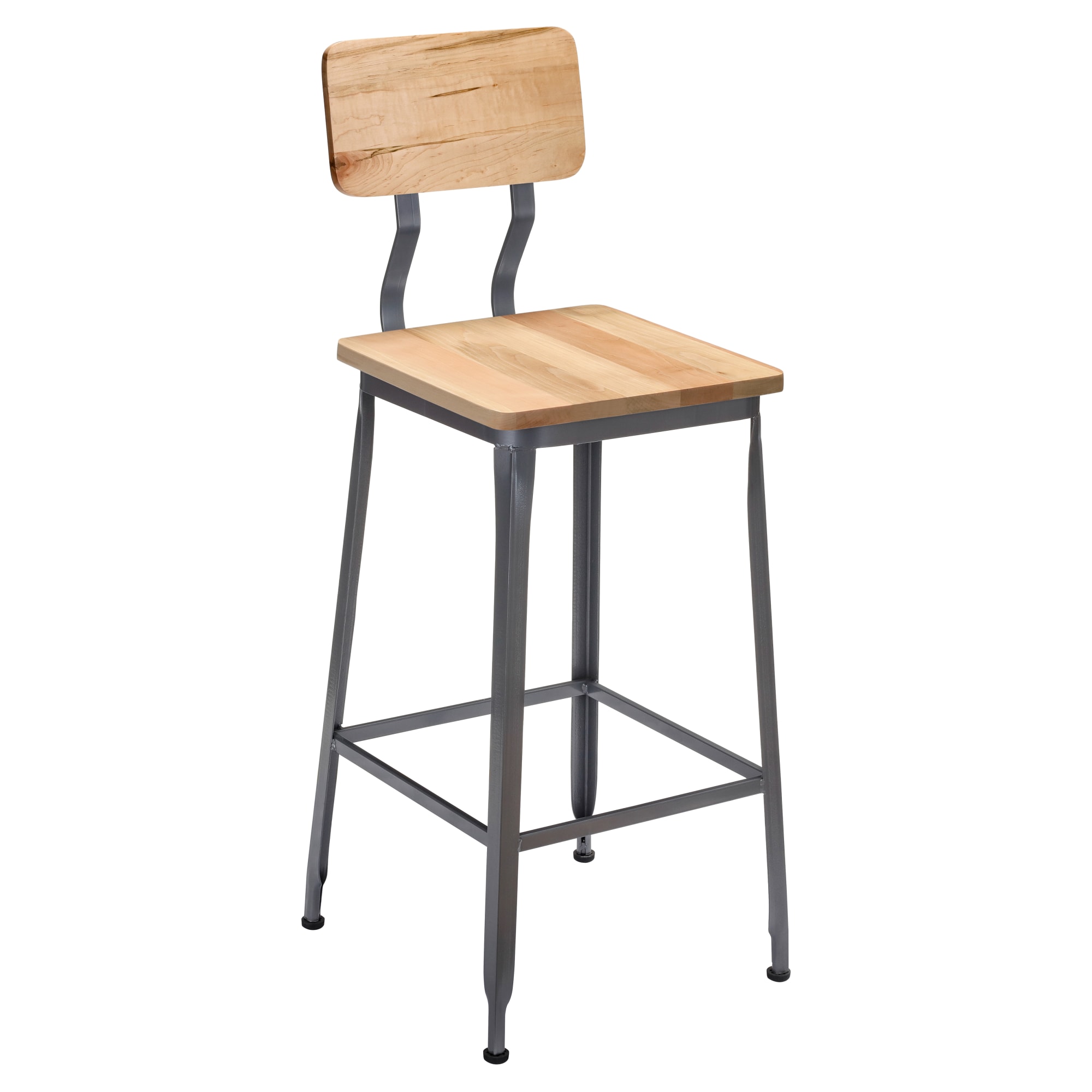This image showcases a tall, bar stool-height chair with a minimalist and industrial design. The chair features a sturdy metal base comprised of four gray, tapered legs, each capped with a black rubber foot to prevent sliding. Connecting the legs near the bottom is a square metal crossbar, providing additional stability. The seat and backrest of the chair are made from natural butcher block wood, potentially maple, exhibiting the character of the wood with visible knots and color variations. The rectangular wood backrest is supported by two metal bars extending from the seat, offering ergonomic support. Set against a completely white background, the chair’s simple yet functional design is highlighted, emphasizing its clean lines and lack of decorative elements.